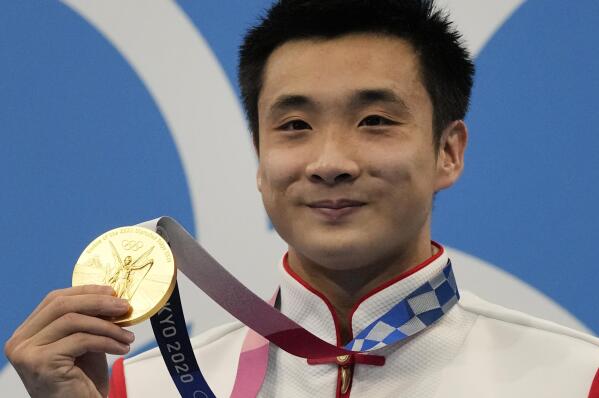This photograph captures an Asian athlete, likely of Chinese descent, who has triumphed at the Tokyo 2020 Olympics by winning a gold medal. He is smiling modestly, with a closed mouth, conveying genuine happiness—the crinkle of his eyes further emphasizing his satisfaction. The athlete is dressed in an official white jacket that features red trim and a gold button clasping it at the neck. His hair is medium length and slightly spiky.

In his right hand, he proudly holds a large gold medallion adorned with the image of a winged angel and the Olympic rings above, with various other inscriptions. The blue ribbon, which features white checkered accents, bears the words “Tokyo 2020.” Behind him is a light blue backdrop featuring the iconic Olympic ring logo partially visible.

This detailed composition effectively highlights the athlete’s joy, his attire, the distinctiveness of the medal, and the significance of his achievement at the prestigious event.